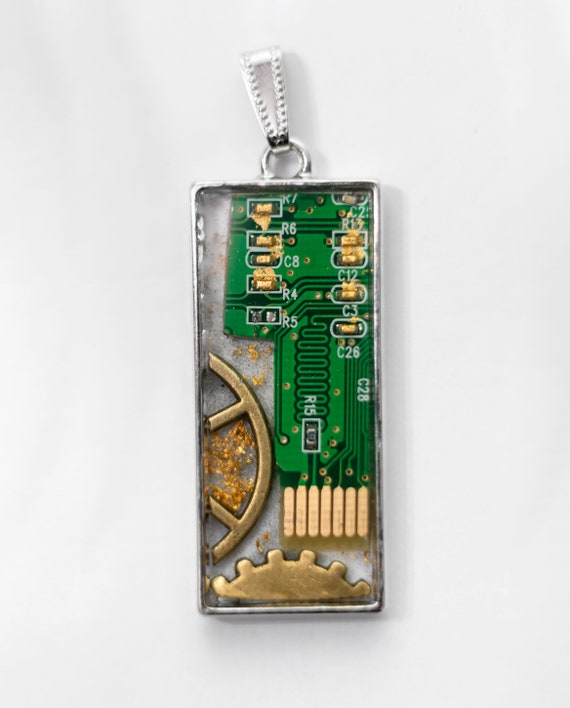This photograph showcases a distinctive piece of jewelry designed to be worn as a pendant. Encased in a transparent protective cover, the centerpiece is a rectangular segment of a green circuit board, adorned with small gold contacts labeled with identifiers such as R6, C8, R4, and others, suggesting places where buttons or components might once have been connected. The bottom of the circuit board features a gold-plated area, likely a connector slot. Additionally, the case contains a cutout of a metal gear at the bottom embellished with brass shavings and a solid metal wheel on the left side, both contributing to a steampunk aesthetic. Gold glitter is scattered throughout the enclosure, adding a touch of shimmer. The pendant is housed within a silver-toned casing, topped with a loop and clasp, allowing it to be affixed to a chain or string and worn as a necklace.